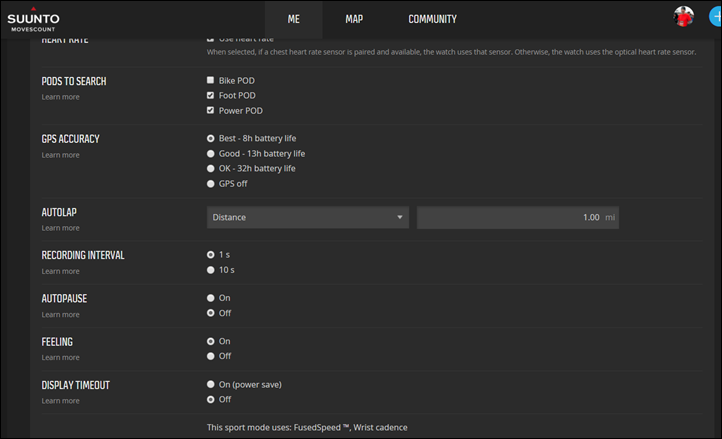This image is a screen capture from a computer monitor displaying an interface of an online application named "Suunto." The application screen features a dark gray background with all text and buttons in white for high contrast. In the upper left corner of the screen, the title "Suunto" is prominently displayed, spelling s-u-u-n-t-o. Directly beneath this, the words "Movies Count" are visible. 

On the left side of the screen is a list of various functional options, including "Pods to Search," "GPS Accuracy," "Auto Lap," "Recording Interval," "Auto Pause," "Filling," and "Display Timeout." These functions are organized in a vertical menu for easy navigation.

At the very top of the screen, centered, are additional navigation tabs labeled "Me," "Map," and "Community." These tabs provide access to different sections of the application, facilitating user interaction and navigation within the app. The overall layout is clean and user-friendly, designed for efficient use and accessibility.